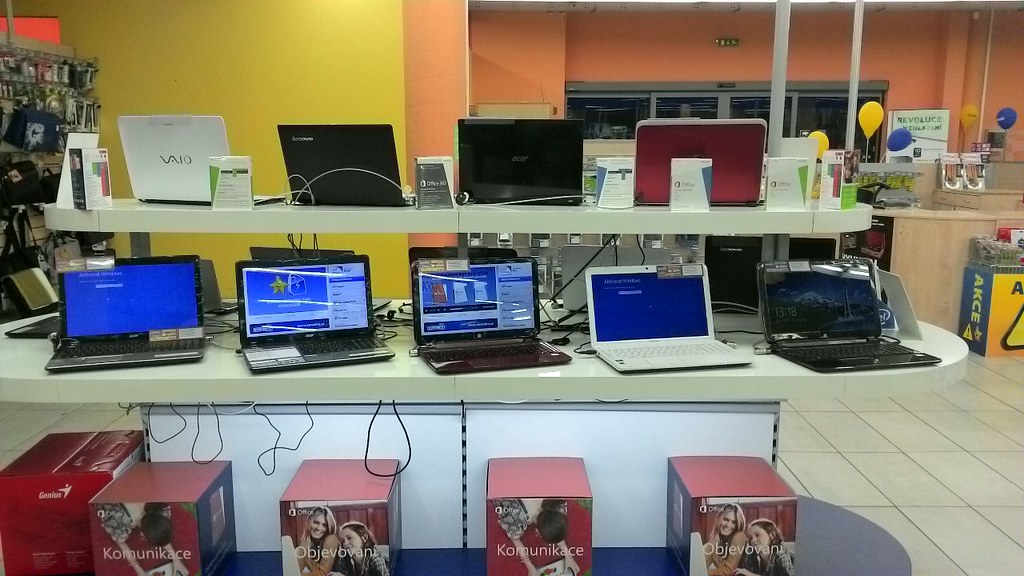This detailed color photograph captures a brightly lit retail store specializing in electronics, particularly laptops. In the foreground, there is a prominent three-tiered white display shelf showcasing a variety of open and powered-on laptops. The display is neatly organized with a striking arrangement of laptops—five on the middle shelf, consisting of four black and one white, and four on the top shelf featuring a white, two black, and a distinctive burgundy red laptop. The screens of these laptops range from blue to displaying specific software interfaces.

Between these laptops on the second shelf, various boxed software including Microsoft Office is prominently placed. Below the display, five striking red cardboard boxes with images of women and foreign lettering are neatly lined up, serving as an advertisement and additional storage. 

In the background, the store's walls transition from a yellow on the left to a tangerine orange on the right, adding vibrancy to the scene. On the far right, red and blue balloons are visible, likely highlighting a promotion or special event. To the left, an accessory wall is adorned with a variety of phone cases, mouse pads, and other electronic accessories. The grey tiled floor and additional shelving units further emphasize the well-organized and comprehensive range of electronic goods available at this store. A faint view of a beige wooden desk cluttered with items and a grey glass sliding door in the distance completes this bustling store environment.